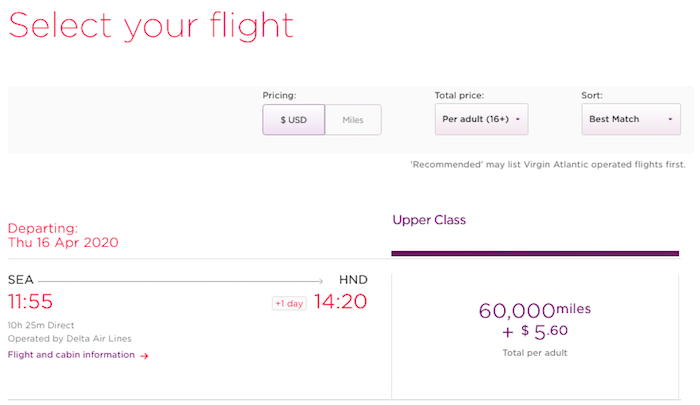The image displays detailed flight booking information on a webpage. At the top left corner, there is a prominent red heading that reads, "Select Your Flight." Below this heading is a light gray bar spanning the width of the page, containing three rectangular options. The first option, labeled "Pricing," is set to U.S. Dollars with the alternative option of selecting miles, though this is currently not highlighted. The second option, "Total Price Per Adult 16+," displays a clickable link with a dropdown menu. Similarly, the third option, "Sort," shows "Best Match" with another clickable dropdown menu.

Further down, there is a star icon followed by a note stating, "Recommended—may list Virgin Atlantic operated flights first." On the bottom left corner, "Departing Thursday, April 2020" is highlighted in red. Below this, "SEA ➔ HND" indicates the flight route from Seattle (SEA) to Tokyo Haneda (HND). Under "SEA," the departure time is listed as "11:55 AM," and under "HND," the arrival time is "14:20," with a note in a small rectangular box displaying "+1 Day." The flight duration is noted as "10 hours, 25 minutes direct," operated by Delta Airlines. A purple link labeled "Flight and Cabin Information" is also present.

To the right-hand side, there is a rectangular box labeled "Upper Class," with purple text inside it stating, "60,000 miles plus $5.60 total per adult."